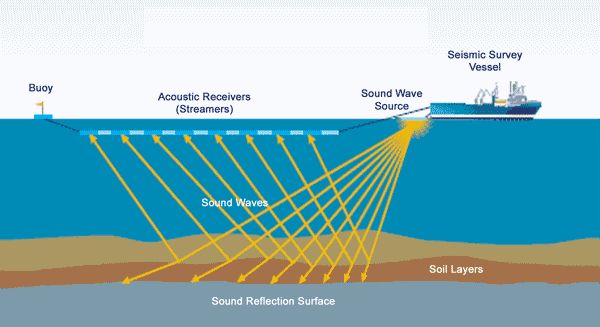The image is a detailed diagram of a seismic survey process carried out by a seismic survey vessel. The diagram is enclosed in a rectangular box displaying four distinct layers of color representing different geological sections. The top layer is turquoise blue, denoting the water surface, below which a light tan section indicates the upper soil layers. This transitions to a darker tan section and then to a gray bottom layer, which is labeled as the sound reflection surface.

On the right side of the image, the seismic survey vessel floats on the water's surface, labeled clearly. From the vessel's bottom, yellow arrows labeled as sound wave sources spread out into the blue water, forming a triangular shape. These sound waves travel down to the brown soil layer and reflect back upwards. The returning sound waves are intercepted and collected by a horizontal line made up of alternating light and lighter blue segments, labeled as acoustic receivers or streamers.

These acoustic receivers are connected to a buoy located in the upper left corner of the image, depicted as a small blue cup with a yellow flag. The various parts of the diagram, such as the vessel, sound waves, acoustic receivers, and soil layers, are precisely labeled to illustrate the function and process of the seismic survey.